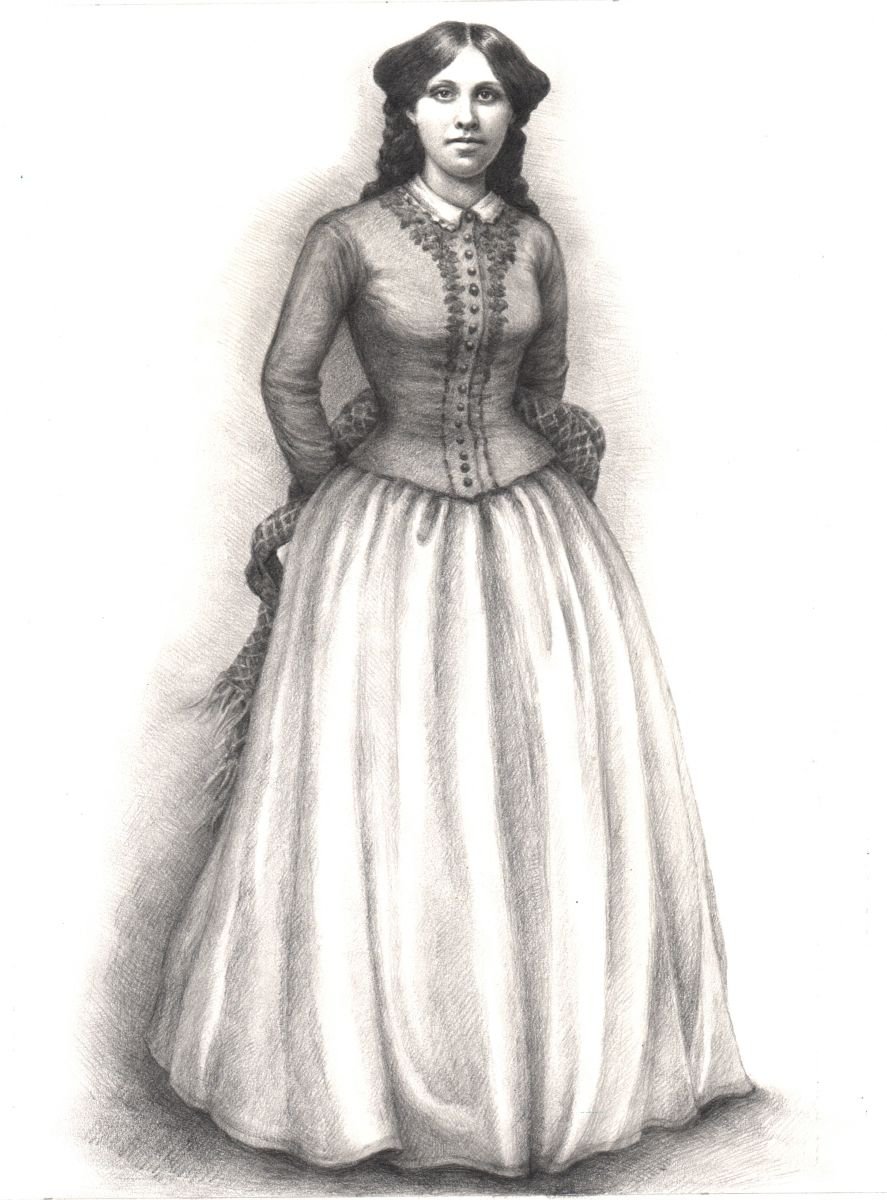This detailed, realistic charcoal or pencil sketch portrays a woman standing at the center of the composition against a stark white background. She is donned in an ensemble that hints at late 19th-century fashion. Her attire features a darker gray, full-sleeved blouse with intricate embellishments along the seams and buttoned down the middle to the waist. This blouse seamlessly transitions into a flowing, voluminous white gown adorned with frills. The gown extends all the way to the floor, obscuring her feet, and accentuates her cinched waistline. The woman’s dark hair, almost black, is poofy and styled into a curly braid that drapes down her back. A shawl or veil with a checkered plaid pattern, exhibiting threads of fabric at its ends, is held behind her. She gazes directly at the viewer with a slightly smiling, straightforward expression, her dark wide eyes conveying a sense of calm. The rendering of her features is so meticulous and soft that the sketch exudes a lifelike quality, similar to a black-and-white photograph.